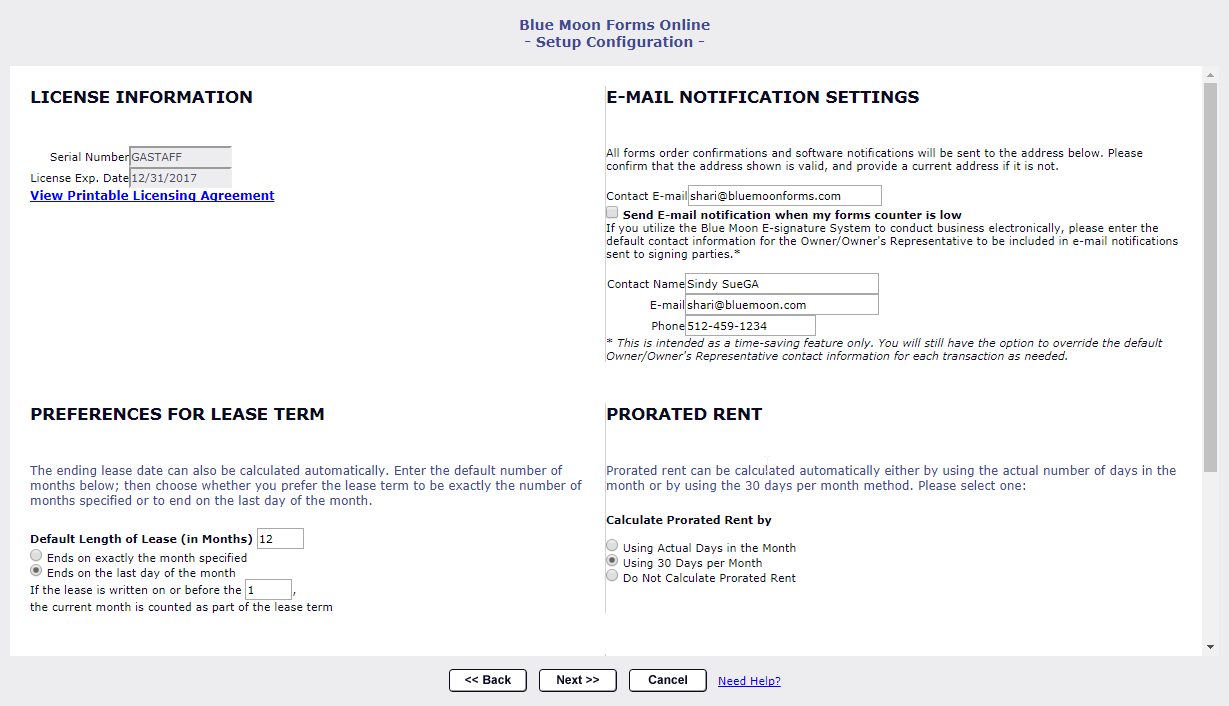**Detailed Caption:**

This screenshot captures the "Blue Moon Forms Online Setup Configuration" page. At the top of the image, a gray banner features the central title. Beneath this banner, within a white section, several important settings and information are displayed.

The first section titled "License Information" includes:
- Serial Number: G-A-S-T-A-F-F
- License Expiration Date: 12-31-2017
- A link to view the Printable Licensing Agreement

Following this, the "Preferences for Lease Term" segment allows users to input lease term preferences. It provides instructions stating, "The ending lease date can also be calculated automatically. Enter the default number of months below, then choose whether you prefer the lease term to be exactly the number of months specified, or to end on the last day of the month." Options include:
- Default length of lease in months: 12
- Ends on exactly the month specified
- Ends on the last day of the month (this option has been selected)
An additional note clarifies, "If the lease is written on or before the 1st, the current month is counted as part of the lease term."

In the "Email Notification Settings" section, the configuration ensures:
- All forms, order confirmations, and software notifications will be sent to "shari@bluemoonforms.com"
- Users must confirm the displayed address is valid and update if necessary
- An option to send email notifications when the forms counter is low

For those using the Blue Moon eSignature system, there's an area to enter the default contact information for the owner/owner's representative. This contact information will be included in email notifications sent to signing parties. The note emphasizes this feature is designed to save time but can be overridden for each transaction.

The "Prorated Rent" section provides choices for calculating prorated rent:
- By using actual days in the month
- Using 30 days per month (this option has been selected)
- Do not calculate prorated rent

At the bottom of the page, navigation buttons include "Back," "Next," "Cancel," and a "Need Help?" link.